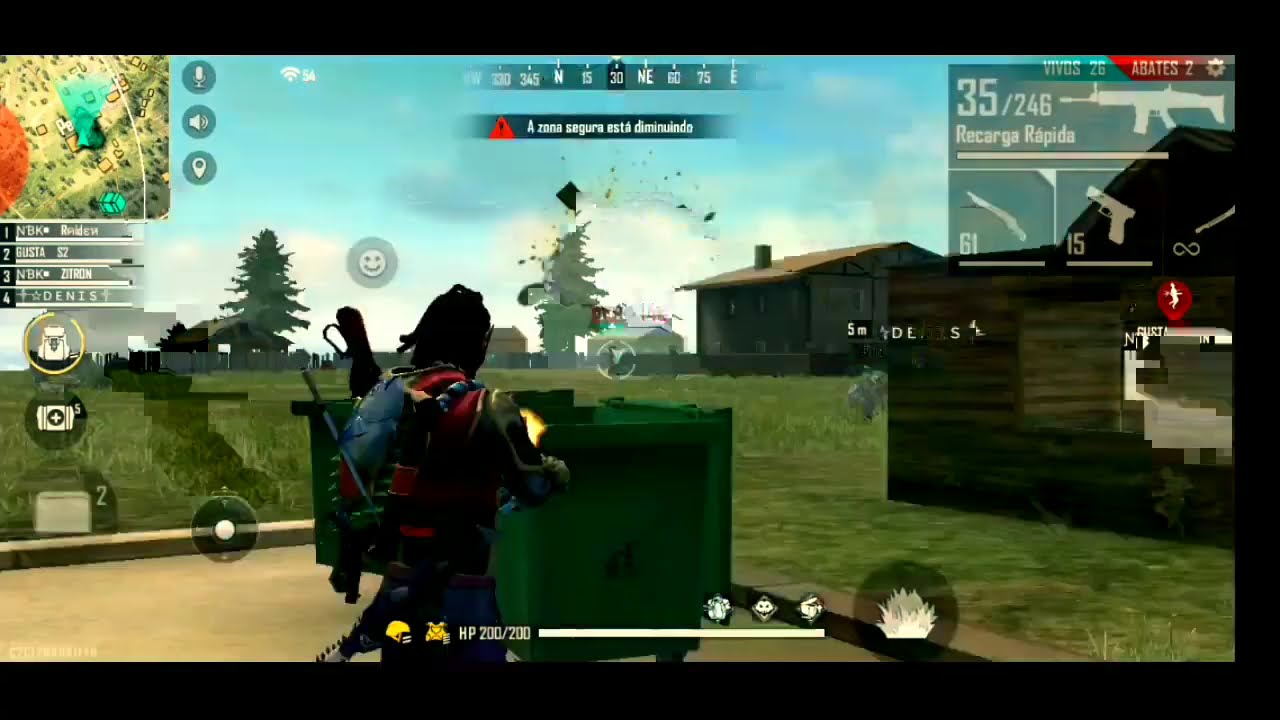In this detailed scene from a first-person shooter video game, a player character is crouched behind a large, green, wheeled dumpster, facing away from the camera. The character appears to be consulting a map while holding a weapon. The surrounding environment features lush green grass and a clear blue sky with a hint of white along the horizon. Two trees stand in the distance against the backdrop of what looks like farmland, including a barn and additional brown structures to the right, possibly storage buildings.

Superimposed on the image are various game interface elements. In the top left corner, a small map displays the terrain. The top right corner features an inventory menu showcasing three different guns and ammunition details, with specifics like "35/246" and "recharge rapids" visible. A list of numbers from one to four appears on the screen, possibly indicating rankings or objectives. Below this, on the bottom of the screen, the player’s health status, "HP 200/200," is displayed alongside other details including a Wi-Fi signal icon marked at 54, and a directional compass indicating orientation, such as north or northeast. Additionally, a smiley face icon and a circular element are seen floating above the player.

In the foreground, the player stands on a dirt path bordered by concrete. A pack is strapped to the character’s back, and gunfire is visible in front of the dumpster, suggesting active engagement in combat.